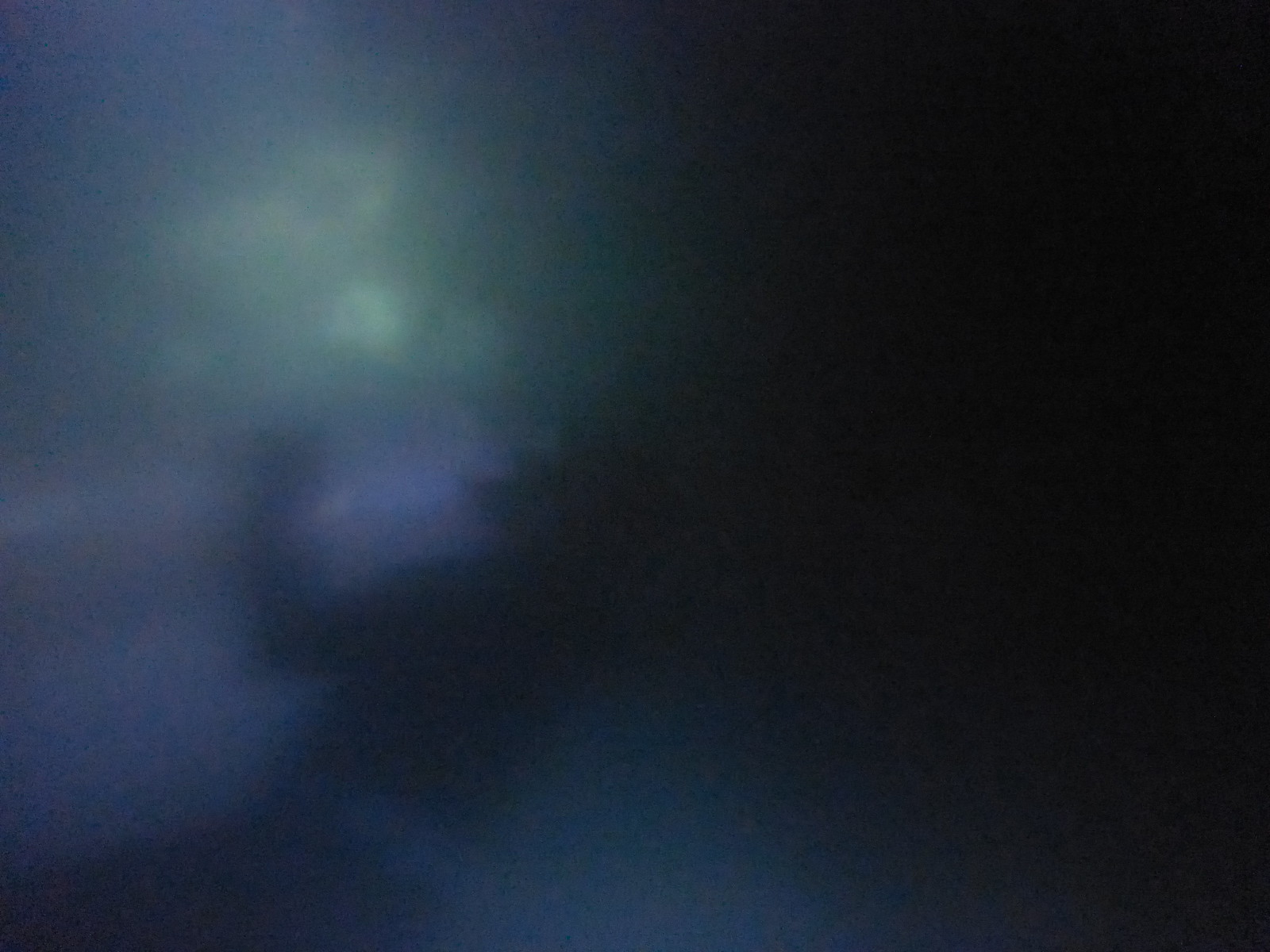In the depths of the ocean, an underwater scene unfolds in a haunting blend of darkness. The image is a symphony of darkish grays, blacks, and deep blues, creating an almost murky haze that shrouds the environment in mystery. The ambiance is one of profound isolation, immersing the viewer in the deep, deep part of the ocean where light barely grazes the surroundings. 

In the far distance, a faint, blurry light pierces through the dense water, hinting at the distant sun struggling to break through the ocean's depths. This subtle glow offers a glimmer of hope and adds an ethereal quality to the scene. 

In the foreground, a shadowy silhouette of a lone human figure is faintly discernible, their presence adding an element of human vulnerability and intrigue to the vast, uncharted underwater world. The figure's form is indistinct, blending almost seamlessly with the shadowy and mysterious deep-sea environment. 

This evocative image captures the essence of the unknown and the isolation of the ocean's deepest parts, inviting the viewer to ponder the mysteries that lie beneath the surface.